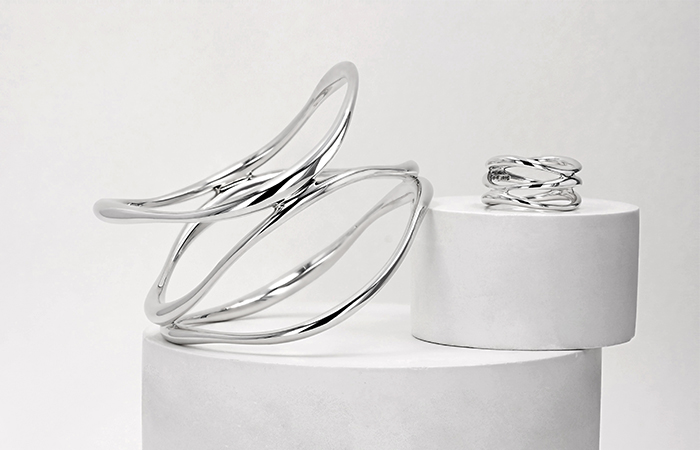The image features a modern, abstract sculpture ensemble against a light gray, almost white background. Central to the composition is a large, cylindrical white base resembling a solid, giant marshmallow. Perched off-center to the right of this base is a smaller, similar white cylinder, slightly overhanging the edge. On top of this smaller cylinder sits a shiny, silver metallic sculpture composed of three interconnecting rings, evoking the appearance of spirals. To the left, angled and leaning against both the large and small white cylinders, is a larger silver sculpture resembling an abstract, curved ringed shape with a central arc, almost like a stylized football with a scoop on top. The juxtaposition of the sleek, reflective metallic structures with the solid white cylinder bases creates a striking contrast within the minimalist setting.